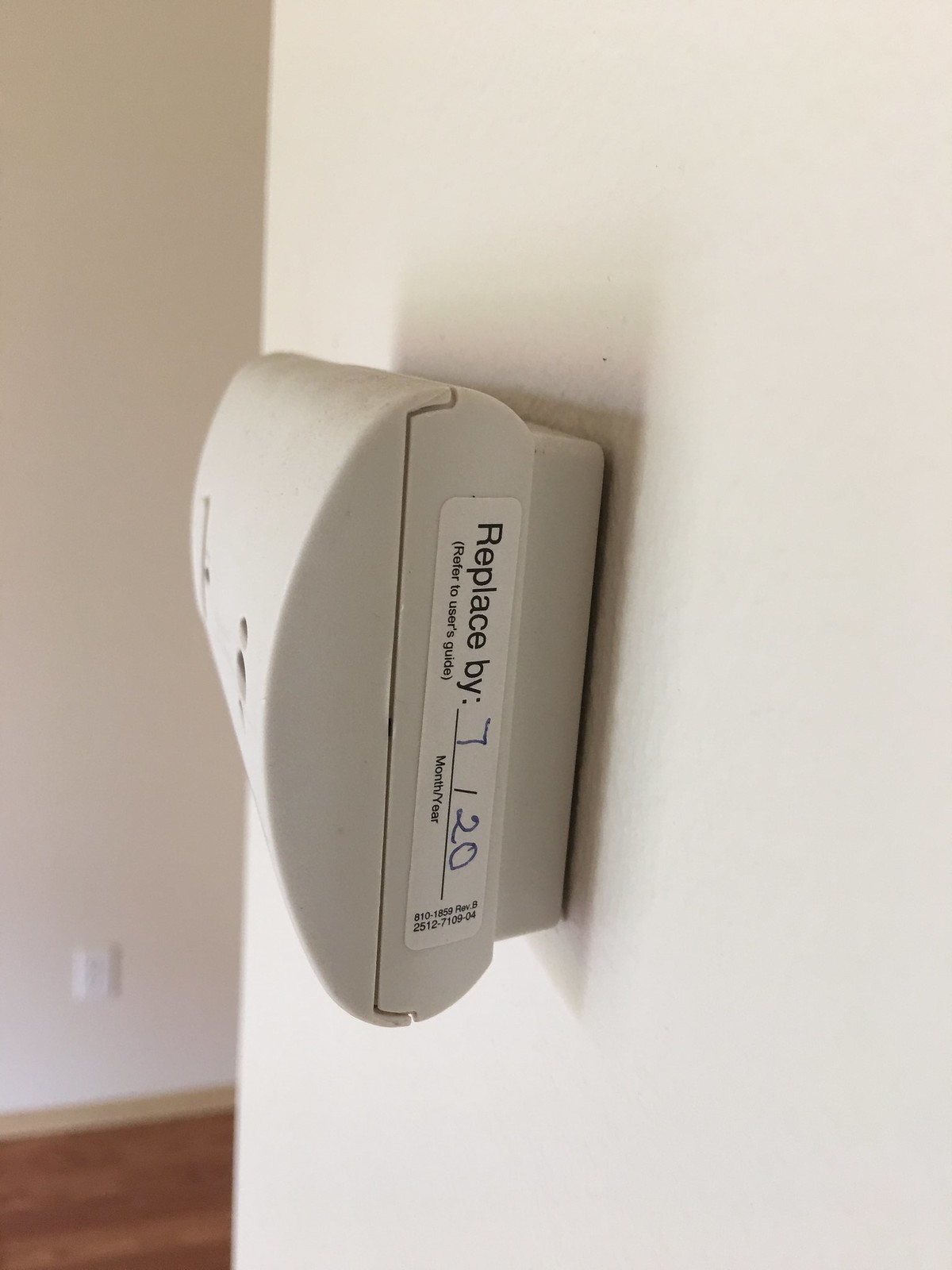The image depicts a room with pristine white walls and a wooden floor. The composition reveals two walls that form a hallway between them; the wall on the left side of the picture extends towards the back, while the other wall runs in the background. On the back wall, there is an electrical outlet. Prominently featured on the wall in the foreground, a white plastic dispenser is mounted. The dispenser, which is slightly rounded at the front, appears to be flush with the wall but protrudes a bit. Its design suggests that the front panel could be detached or lifted for access. Small holes are visible on the front of the dispenser, casting shadows on the adjacent white wall. On the side of the dispenser facing the camera, a sticker is affixed. The sticker reads "Replace by," followed by a blank line intended for a date and "Month/Year 720." Below this, in parentheses, it instructs "Refer to user's guide." The sticker also features some other miscellaneous numbers at its bottom.